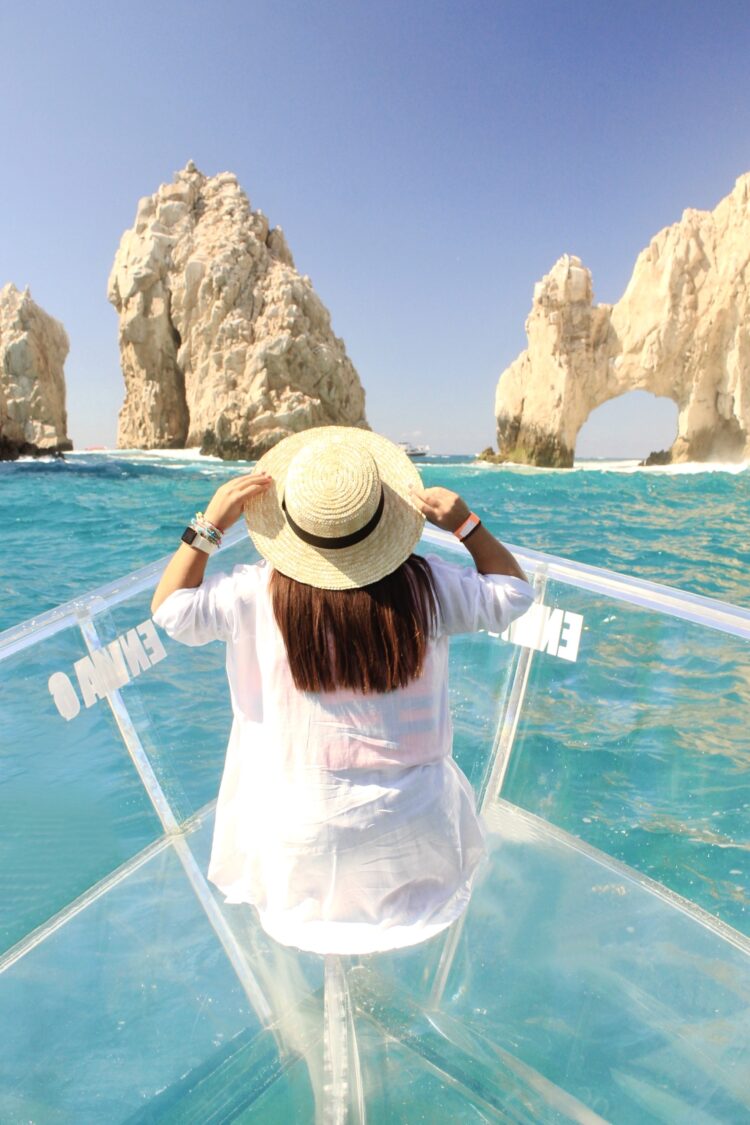The photograph captures a woman with long brown hair, wearing a white shirt and a white, floppy sun hat. She stands at the front of a glass boat, which creates an illusion of her hovering over the pristine, deep turquoise water. The boat features some reversed text on its front, adding to the mysterious ambiance. She is accessorized with a watch and multiple bracelets. The serene, cloudless sky above is a bright blue, seamlessly merging into the stunning water below. In the background, striking white and sandy-colored rock formations rise majestically from the water. The formation on the left and in the middle appears solid, while the one on the right resembles a cathedral archway large enough to sail through. At the base of these rocks, hints of moss add a touch of vibrant green to the scene. The overall effect is one of tranquil beauty, highlighting the woman as she gazes out over the breathtaking landscape.